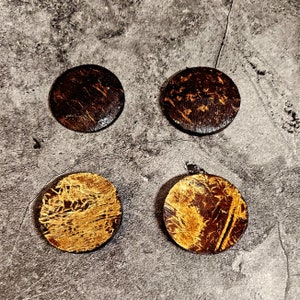The image showcases four distinct round stones set against a varied gray stone-like background, which has an uneven, cracked appearance. The stones are aligned in the center of the frame, resembling the four dots on a die. The two stones at the top are a dark brown color with subtle variations: the left one has light tan lines running across its surface, while the right one features small tan blotches roughly the size of a pinky dabbed in light gray-tan paint. The stones on the bottom are slightly larger and predominantly showcase gold and yellow hues with intricate scribble-like patterns. The left bottom stone is almost entirely covered in this gold paint, leaving just the edges with brown spots about the size of a pea. The right bottom stone exhibits a more uneven distribution, with one half featuring yellow and gold textures intermixed with gray, while the other half remains mostly brown, accented by a few thin gold stripes and squiggly lines. The overall composition hints at the artificial cut and sheen of the stones, adding a touch of deliberate artistry to a naturally inspired setting.